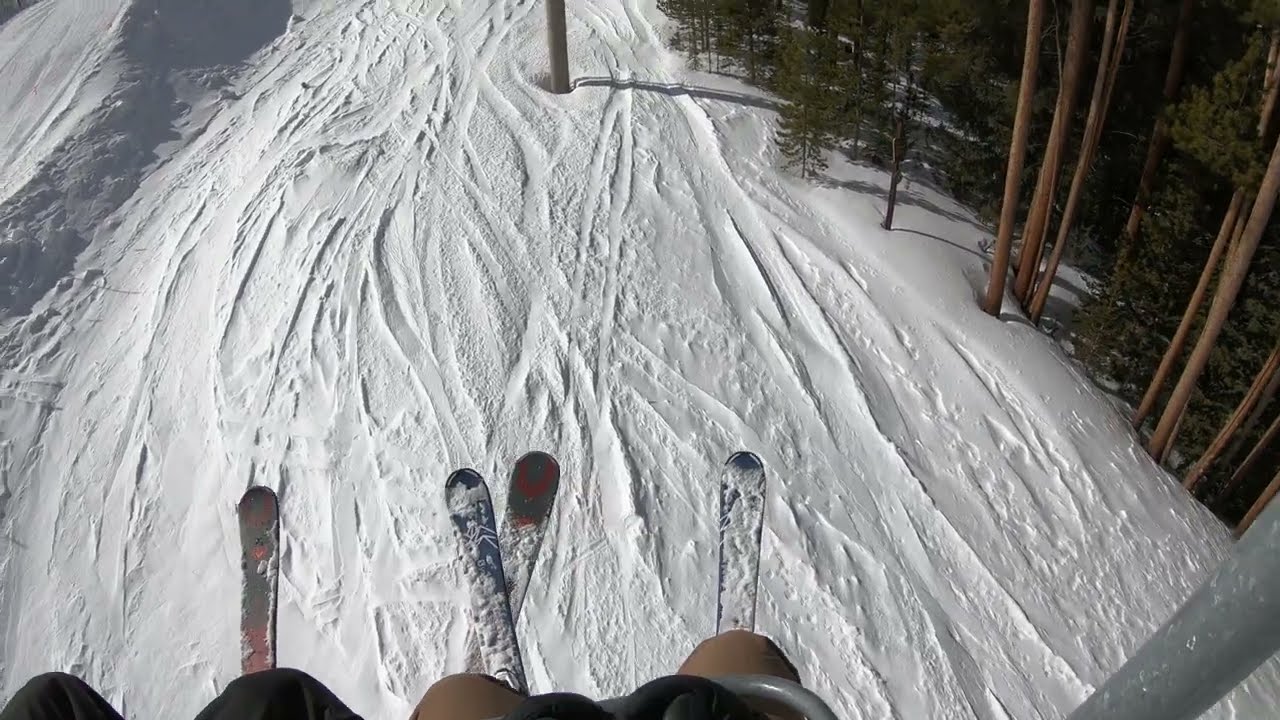This photograph, taken from the vantage point of riders on a ski lift, captures an aerial view of a snowy ski resort scene. In the foreground, you see four skis and the knees of two skiers, partially obscured by a gray lift bar. The ground below is blanketed in white snow, crisscrossed with narrow, skinny tracks from previous skiers. On the right side of the image, a line of trees with brown trunks and some evergreen foliage marks the edge of the ski path. To the left, a snow-covered incline rises up, creating a natural trench. Silver poles, part of the ski lift infrastructure, can be seen intermittently across the scene. The photograph appears to be taken in mid to late afternoon, suggested by the steep angles of the shadows cast on the snow.